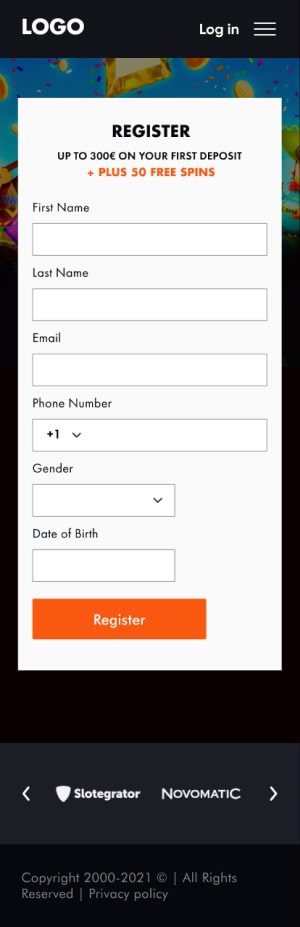This tall and narrow image presents a structured promotional page. At the top, a black banner features the word "LOGO" in bold, white capital letters situated in the top left-hand corner. To the right, the banner displays "LOG IN" followed by three horizontally stacked white lines.

The image's midsection bursts with vibrant colors, primarily blue and gold, reminiscent of confetti swirling in the air. Overlaying this festive backdrop is a prominent registration bar boasting an offer: "Register up to 300 EUR on your first deposit plus 50 free spins." Below this enticing message are fields for entering personal information: first name, last name, email, phone number, gender, and date of birth. The section is capped with a conspicuous orange "REGISTER" button. It's noted that the fields are currently blank.

Below the registration section, a black background transitions to a gray banner featuring two sets of opposing white arrows pointing left and right. Between the arrows are two labels: "Slot Greater" and "Novomatic," both in white text.

At the very bottom of the image, on another black banner, the text reads: "© 2000-2021, All rights reserved, Privacy Policy," hinting that the "Privacy Policy" might be a clickable link for more detailed information. The recurring "LOGO" suggests it is the brand name of the company.